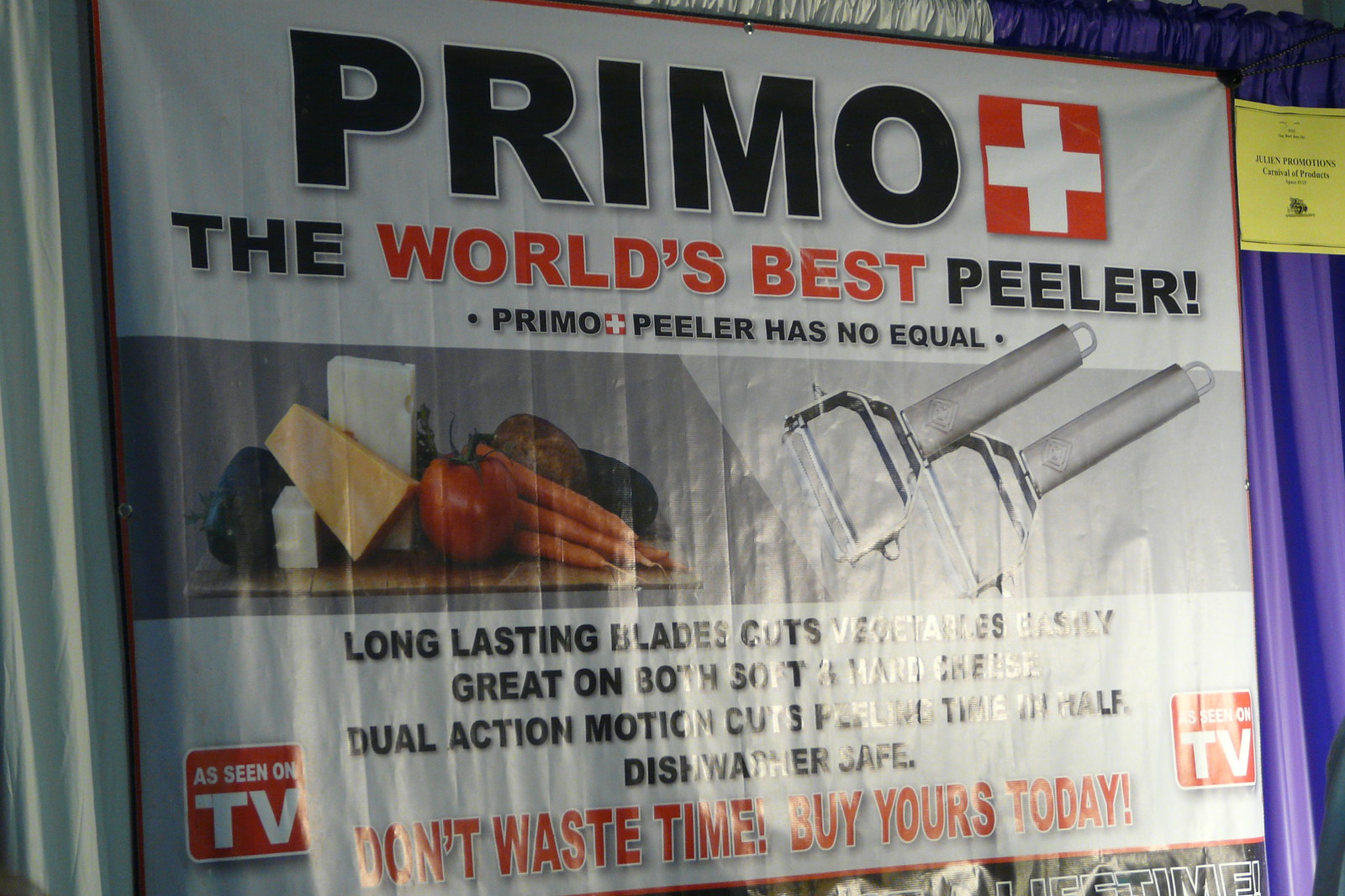This image is a large, glossy banner advertisement, likely from a magazine, featuring a detailed promotion for the "Primo Peeler." The advertisement prominently showcases the brand name "PRIMO" at the top in black text, accompanied by a red and white icon resembling the Switzerland flag. Below this, the tagline "The World's Best Peeler" and "Primo Peeler Has No Equal" are clearly displayed. The center of the ad features vivid images of the product: two sleek vegetable peelers positioned side by side, along with a colorful assortment of vegetables and cheeses, highlighting the peeler's versatility. The background has a white base with black and red text detailing the product's features, such as "Long-Lasting Blades," "Cuts Vegetables Easily," "Great on both soft and hard cheese," and "Dual Action Motion Cuts Cutting Time in about half." Despite some words being obscured by glare, phrases like "Dishwasher Safe" can still be seen. At the bottom corners, red squares with white text prominently declare "As Seen On TV," and a final call to action at the bottom urges, "Don't Waste Your Time, Buy Yours Today."